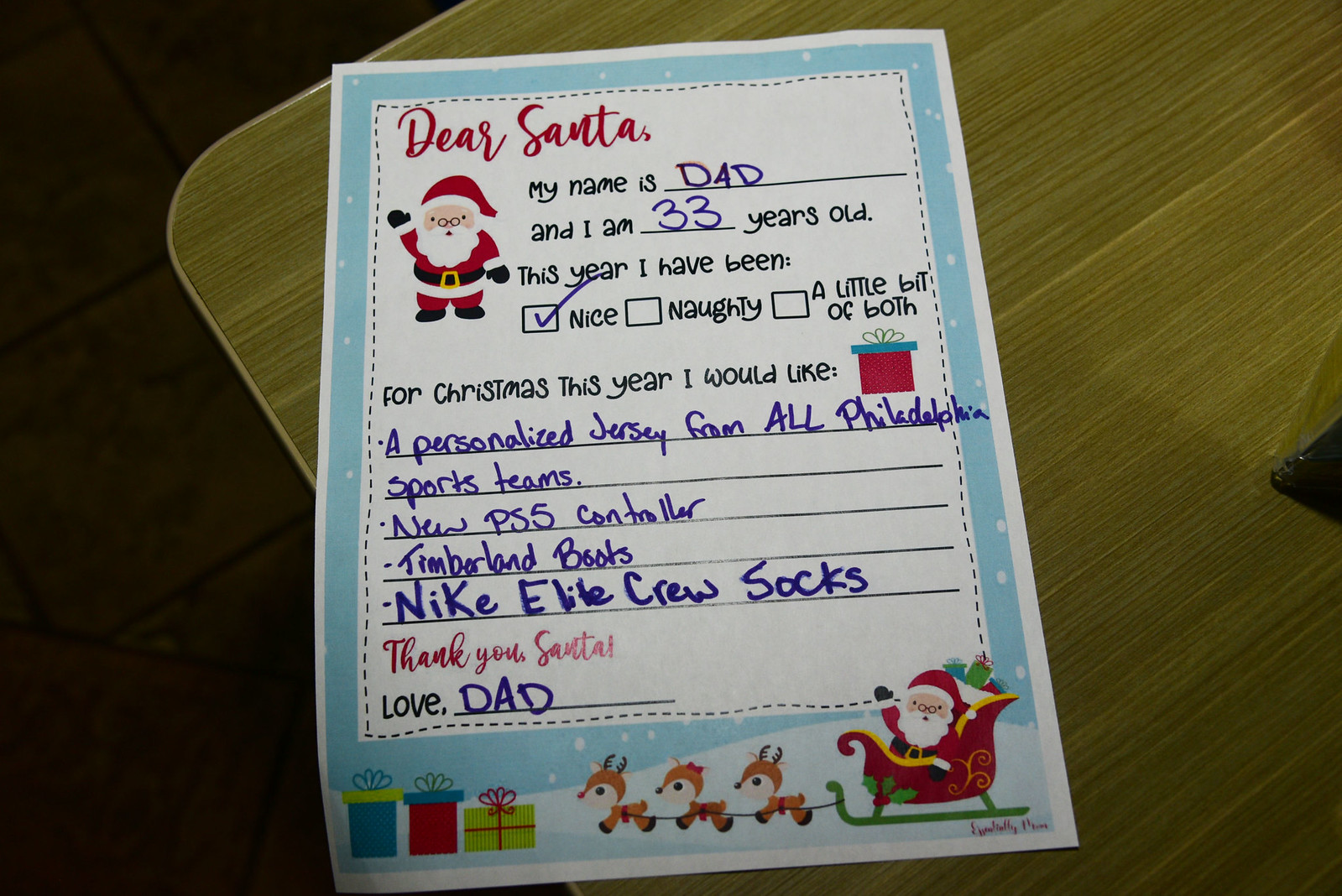The image captures a detailed view of a pre-made letter to Santa, lying on the edge of a brownish-green wooden table with a curved corner, set against a dark-tiled floor. The letter itself features a light blue background adorned with snowflakes and a dotted-line border surrounding the main text area. The letter reads in red cursive, "Dear Santa," followed by fill-in-the-blank prompts pre-printed with "My name is Dad and I am 33 years old. This year I have been," with checkboxes for "nice," "naughty," and "a little bit of both," with "nice" checked off in pen. The letter continues with "For Christmas this year I would like," accompanied by a present icon and lines for listing gifts. The list specified includes: a personalized jersey from all Philadelphia sports teams, a new PlayStation 5 controller, Timberland boots, and Nike Elite crew socks. The form concludes with "Thank you Santa, love, Dad" written in pen. Decorative images embellish the letter, including Santa in his sleigh with three cartoon reindeer, and presents.